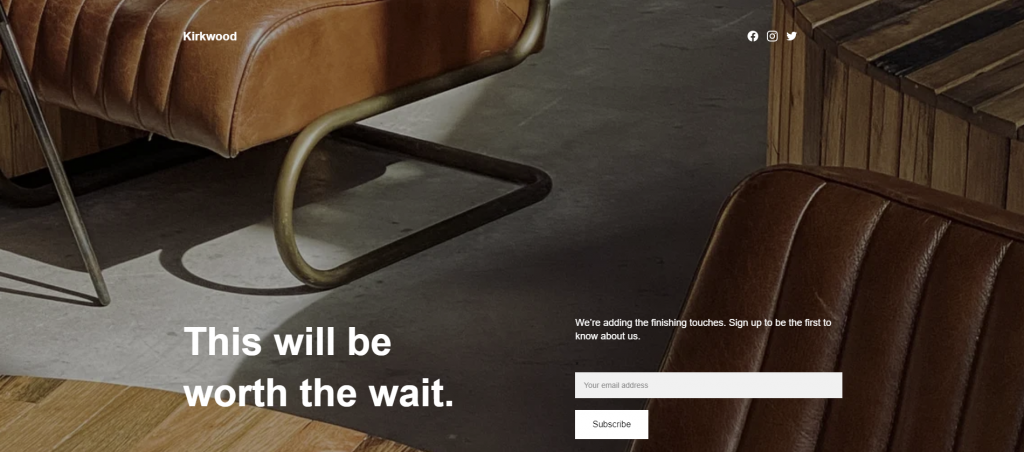The image appears to be a promotional screenshot for the Kirkwood brand, set against an elegantly staged background featuring premium leather sofa chairs positioned on an industrial composite floor. The setting conveys a sense of luxury and modernity, complemented by a rustic wooden crate and possibly a wooden table, suggesting high-quality, carefully curated furniture. The overall ambiance is enhanced by the appealing varnish and rich colors visible in the scene, indicating a premium product line.

In the foreground, the promotion strategically includes clickable icons for Facebook, Instagram, and Twitter, directing viewers to Kirkwood's social media accounts. Prominent white text at the bottom of the image reads, "This will be worth the wait. We're adding the finishing touches. Sign up to be the first to know about us." Below this, a text box invites users to enter their email address, accompanied by a "subscribe" button, encouraging visitors to join their mailing list for updates. The company's approach is intentionally enigmatic, aiming to build anticipation and curiosity without revealing specific details about their offerings.